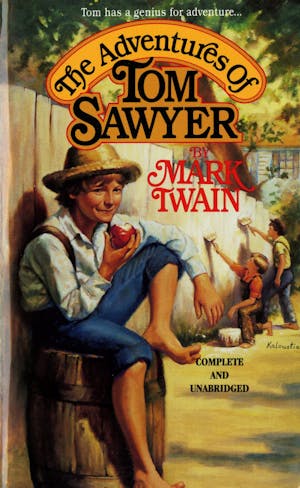This detailed book cover illustration for "The Adventures of Tom Sawyer" by Mark Twain captures the essence of Twain's beloved classic. The top of the cover features a line of white text that reads, "Tom has a genius for adventure..." set against a green leafy canopy. Below this, the title "The Adventures Of" is written in black text over a yellow, orange-tinged background, with "Tom Sawyer" prominently displayed in bold letters. The author's name, "By Mark Twain," stands out in red lettering against the white picket fence that frames the lower portion of the cover. 

Dominating the scene, a young Tom Sawyer is perched on a wooden barrel against the white fence, casually enjoying an apple, with a mischievous grin hinting at his well-known escapades. Tom, identifiable by his straw hat, reddish hair, and fair skin, is dressed in a long-sleeved white shirt with suspenders and blue knee-length pants, his bare feet emphasizing the summertime setting. His left leg is bent at the knee, heel resting on the barrel, while his right leg dangles freely.

In the background to the right, two children are depicted painting the fence. One, possibly a girl, is dressed in brown overalls and a red shirt, while the other, a boy, wears dark gray trousers and a short-sleeved white shirt with suspenders. The text "Complete and Unabridged" sits neatly on the ground beneath them, rounding out this classic cover design which perfectly encapsulates the wit and charm of the original tale.